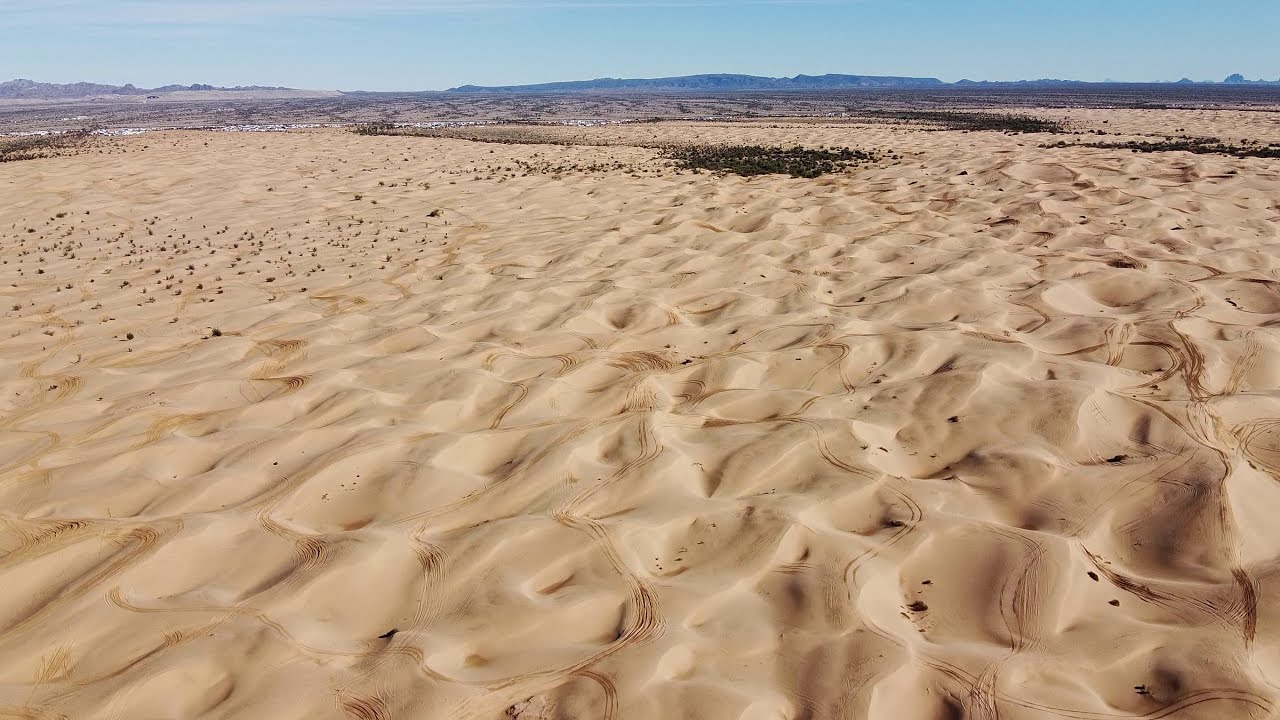This high-altitude photograph captures the vast expanse of a sandy desert, likely located in the Africa or Middle East region. The predominant feature is the light beige sand dunes, which create a mesmerizing pattern of hills and valleys, resembling waves. Scattered across the dunes are numerous pits and tracks, possibly tire marks, weaving through the sandy landscape.

Amidst the sand, small black specks dot the scene, potentially indicating either rocks or entire trees, the scale remains ambiguous. As the image extends towards the horizon, particularly to the left, a concentration of these black specks suggests the presence of an oasis, with other similar patches scattered throughout the expanse.

The backdrop reveals a distant low mountain range flanking both sides of the photograph, against a clear blue sky. Sparse green patches, possibly indicating small patches of greenery or trees, break the monotony of the sand. In one area towards the horizon, there might be a blurred indication of buildings or a small civilization, adding a hint of human presence to this predominantly uninhabited desert landscape.